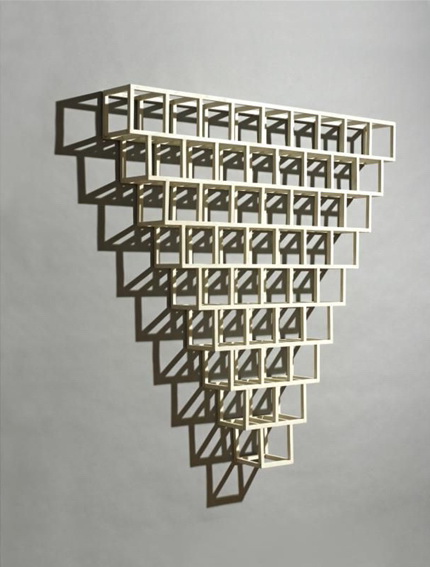The image showcases a modern sculpture attached to a pale gray wall, featuring an intricate upside-down triangular design. This striking piece of art is constructed from rows of white cubes or silver wires, meticulously woven together to form a geometric pattern. The sculpture consists of nine rows, with each subsequent row containing fewer cubes or wires, creating the impression of a downward-pointing triangle. The shadows cast by the lighting enhance the geometric complexity, with a prominent black shadow mirroring the sculpture's triangular form on the wall, adding a three-dimensional effect. The delicate interplay of light and shadow, combined with the repetitive arrangement of the rows, offers a captivating visual experience.